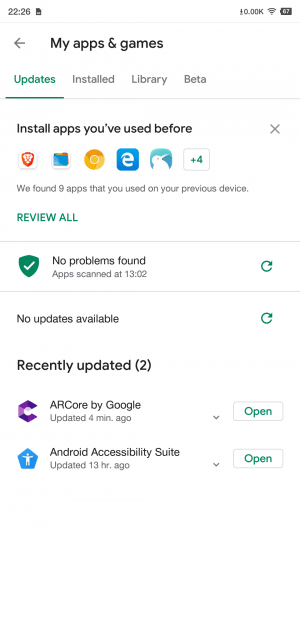A screenshot captures a user's cell phone display, presenting a predominantly white screen. The time is prominently displayed in the upper left corner, reading 22:26, while the far right shows a battery life at 67%. Centered in black text, the header "My Apps and Games" with a back arrow is visible. Below this header, four options appear: Updates (highlighted in bright green with an underline), Installed, Library, and Beta, all in light gray text except for the highlighted Updates.

Further down, the screen features a statement in black text: "Install Apps You've Used Before," accompanied by an 'X' icon on the far right for closing the section. Beneath this, several app icons are aligned horizontally, starting with the Brave browser icon, followed by other unrecognizable icons. Accompanying this display is a note in gray text: "We Found 9 Apps You Used on Your Previous Device." Below this note, a prompt in bright green, capitalized letters asks users to "Review All."

At the bottom of the screen, a green shield icon with a white checkmark indicates "No Problems Found, Apps Scanned at 13:02," followed by additional gray text stating, "No Updates Available."